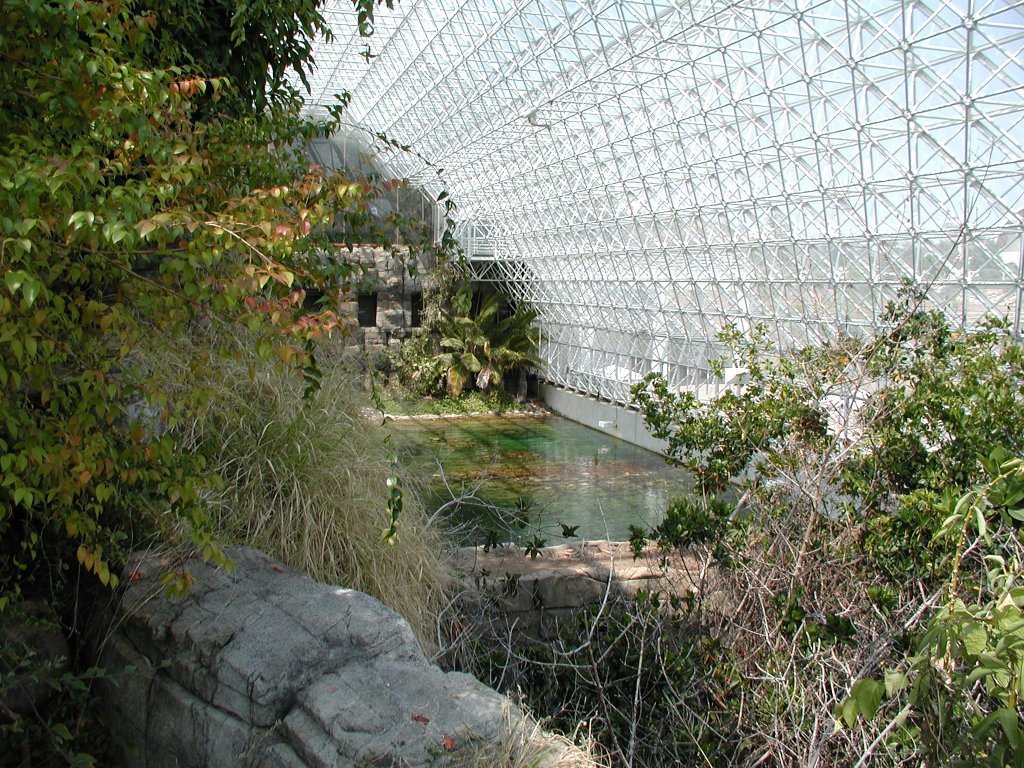This photograph captures the interior of a colossal atrium, possibly part of a museum or conservatory, encapsulated by a glass roof and walls supported by a grid of silver rods arranged in horizontal and diagonal patterns. The atrium is bathed in natural light, streaming through what could be glass or plastic panels. The space is filled with various forms of greenery including trees, shrubs, and bushes, many of which appear to have bare branches interspersed with spots of green foliage. A prominent feature within the atrium is a greenish pool of water, bordered by several stone walls. One of these stone walls, positioned centrally in the image, encloses the pool and is juxtaposed with additional greenery. In the background, more stone structures rise, including a wall with three tall, narrow rectangular windows. The enormous structure stretches out of sight, suggesting an impressive length that could span up to 500 to 1,000 feet. Overall, the intricate design and extensive use of natural elements create a captivating blend of man-made and natural beauty.